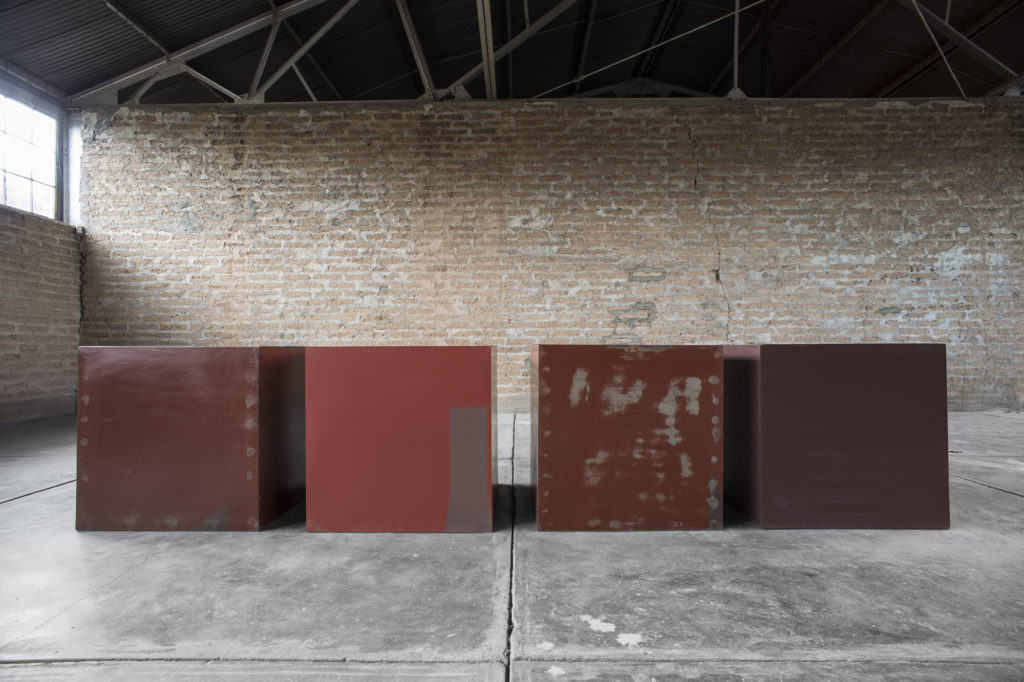In this color photograph taken inside a dimly lit warehouse, four large, worn, metallic-looking boxes are arranged to form the shape of a cube on a gray, cracked concrete floor. The floor consists of panels in varying shades of black, light gray, and white, with noticeable cracks, one of which runs right between the boxes. Each of these boxes are uniform in size and shape, with the box furthest on the left painted a dark amber color, the one next to it a lighter orange with a distinct gray streak, the third box showing patches of peeling orange paint, and the far-right box painted the cleanest, in a very dark amber shade.

The background features a light orange brick wall, inconsistently colored with gouges, black stains, and white patches. These bricks are held together with gray concrete. Looming above the scene is a tin roof supported by steel trusses, reinforcing the abandoned, industrial feel of the environment. In the upper left corner, a window with six panes lets in bright sunlight, casting a glow on the scene. This detailed setup accentuates the stark, rugged atmosphere of the warehouse.